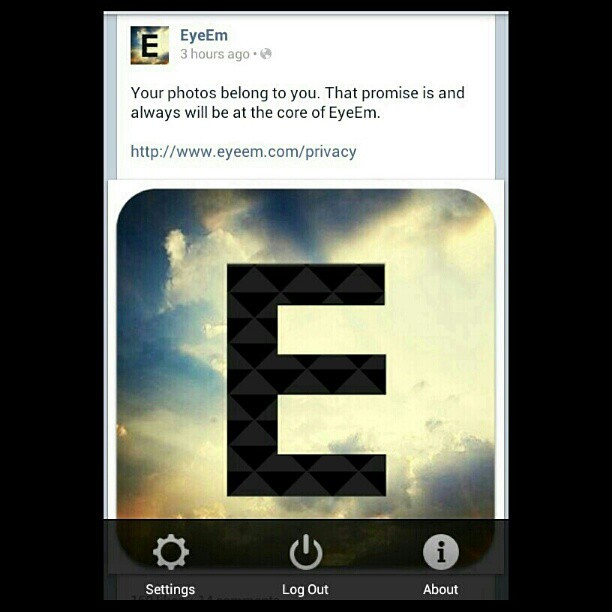This image showcases a central screenshot framed by a solid black background, suggesting it was captured from a social media platform. Dominating the center is a large, stylized letter "E" composed of multiple gray and black triangles, set against a backdrop of yellow clouds and a blue sky. The text at the top reads, "Your photos belong to you. That promise is and always will be at the core of IEM," indicating a privacy assurance from IEM. Below this text, a URL is visible: "http://www.iem.com/privacy." At the bottom of the image, there are icons labeled "Settings," "Logout," and "About," laid out against a white strip. The overall color palette includes black, white, blue, yellow, tan, light blue, and gray. The composition suggests that this screenshot was likely taken from a Facebook post or tweet promoting IEM’s privacy policy.